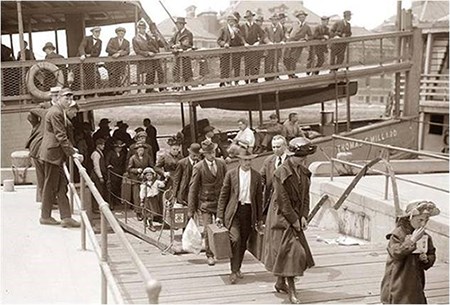The black-and-white photograph captures a bustling scene of people disembarking from a two-level ferry boat named "Thomas Willard" onto a dock. The attire of the individuals in the picture suggests an older time period, with men in suits and women adorned in dresses and hats, carrying suitcases and bags. The dock scene is lively, with a notable presence of observers both on the boat—leaning against the railings on the upper deck—and on the dock, watching the disembarking crowd. A gangplank bridges the boat to the dock, guiding the people to shore, and notably, at the forefront is a small child who appears to be eating something. The image is well-lit and clear, offering a vivid glimpse into a past era.